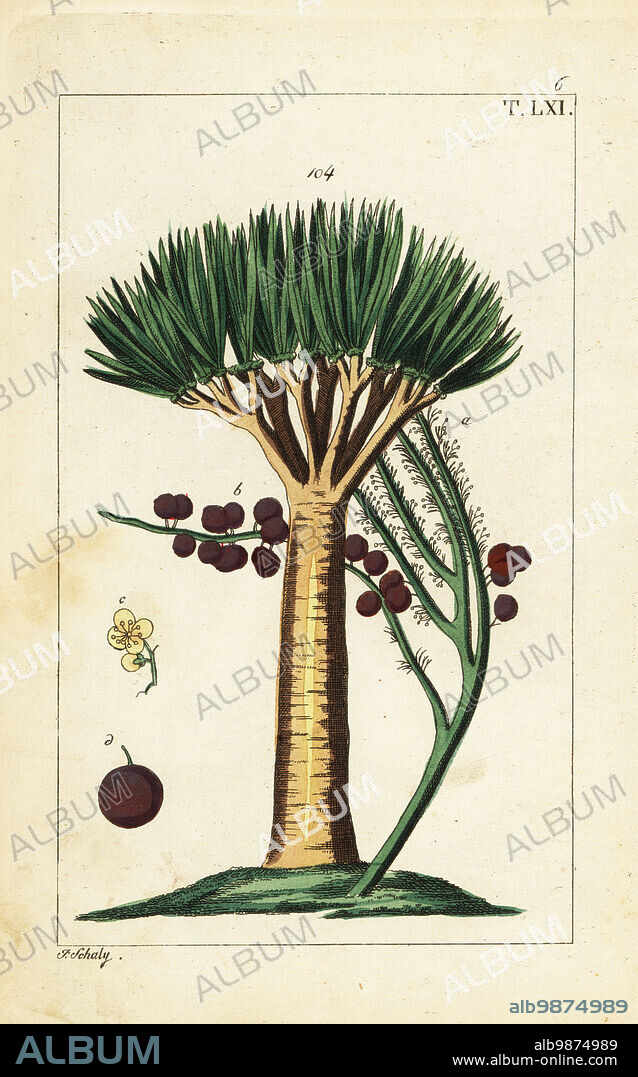In the center of this vertically oriented, rectangular album cover lies a detailed botanical illustration of a tree with a substantial trunk. This trunk extends upward without branches until the top where it fans out into long, pointy green leaves, reminiscent of a palm or coconut tree. Nestled at its base, another plant with slender green branches, delicate hairs, and reddish berries grows out from the green area below the tree. This secondary plant also sports a small yellow flower to the left of the tree. Various letters and numbers label parts of the illustration, including the identifier "T.LXI." at the top and "104" above the plant.

The drawing is framed by an unevenly colored beige border with a thin black outline. At the bottom corner lies the string "ALB9874989," hinting at the image's identifier, alongside the gray text "www.album-online.com." Additionally, a black horizontal bar occupies the bottom, with the gray word "A-L-B-U-M" on the left side. The overall composition includes a watermark pattern repeating the word "ALBUM," securing its online authenticity.